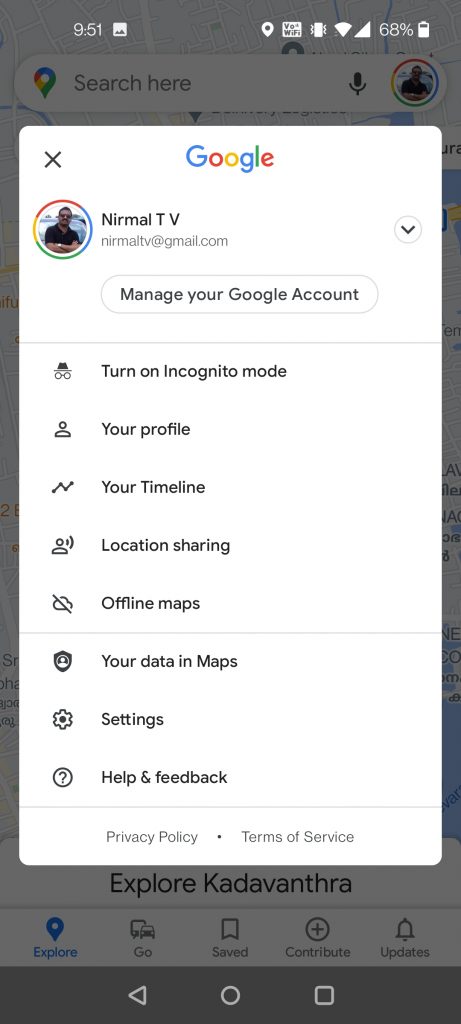This screenshot captures a Google settings page on a mobile device. The background is grayed out with a white overlay at the center, prominently featuring the word "Google" in its iconic blue, red, yellow, and green colors at the top. Beneath this, there's a profile picture of a man wearing sunglasses with his arms crossed. To the right of the profile picture, the text reads "Nermal TV" with the associated email address "NermalTV@gmail.com."

Centered below the profile details is a long oval button labeled "Manage your Google Account." Following this, there are multiple selectable options: "Turn on Incognito mode," "Your profile," "Your timeline," "Location sharing," "Offline maps," "Your data in Maps," "Settings," "Help," and "Feedback." Additionally, links to Google's "Privacy Policy" and "Terms of Service" are present.

The screenshot was taken at 9:51, as indicated in the top status bar, which also shows a location icon, Wi-Fi and cell signal icons, and a battery level at 68%.